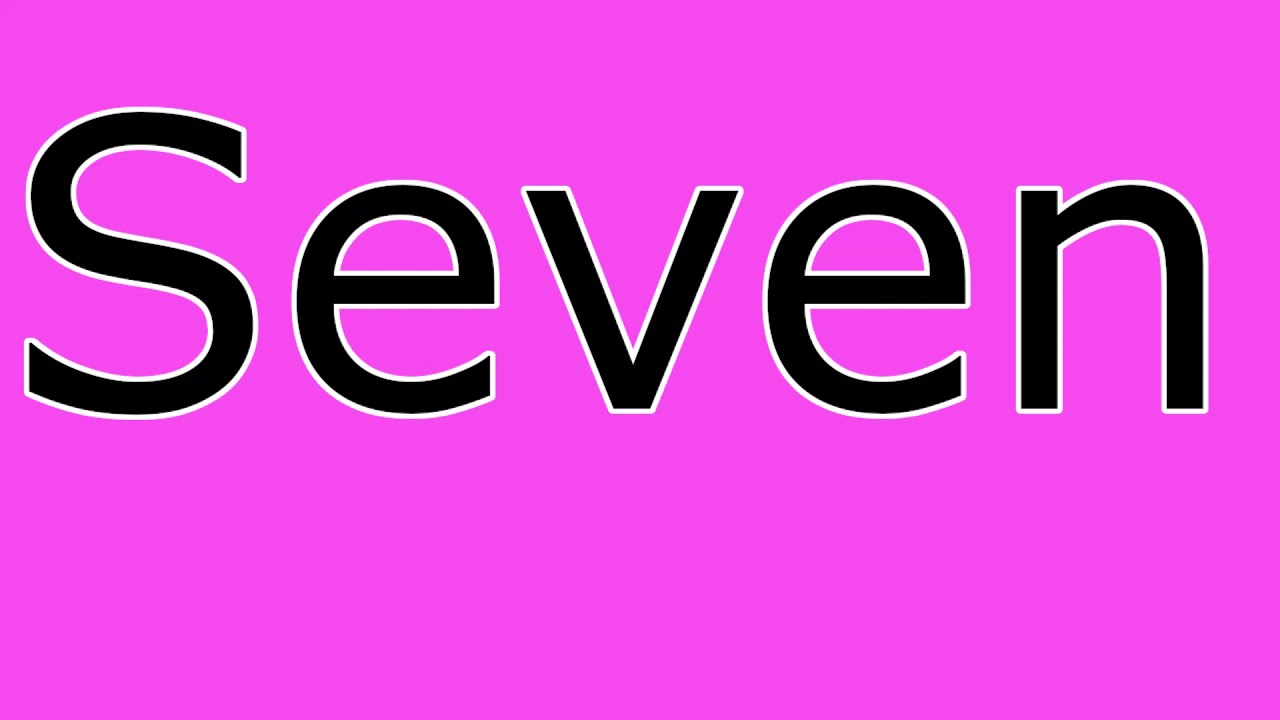This image is a horizontally oriented rectangular graphic with dimensions that are approximately twice as long as they are high. The entire background is a vivid, deep pink hue, tinged slightly with magenta. Prominently occupying the upper half of the rectangle is the word "Seven" displayed in bold, blocky, black text with a thin white outline. The font is plain and sans-serif, with the capital "S" followed by lowercase "e", "v", "e", "n". The spacing between the letters is consistent; however, the text slightly favors the left side, making it appear somewhat off-centered, with the "S" positioned closer to the left edge than the "n" is to the right. The vibrant pink background is uniform throughout, providing a stark contrast to the text.